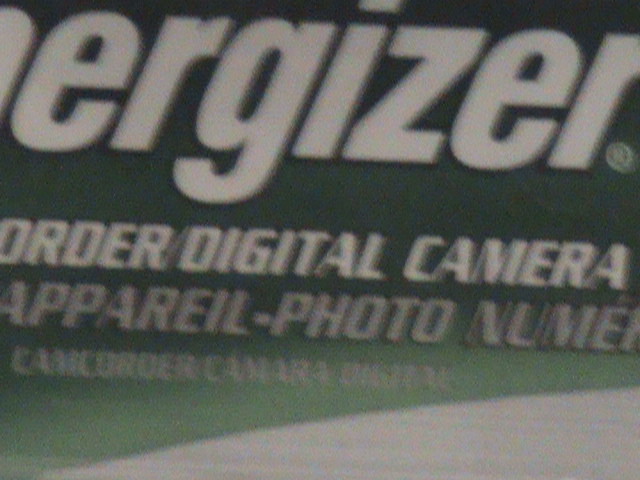A close-up photograph of a green product package with white text. The zoomed-in view partially obscures the words, revealing only fragments such as "er g iz er" at the top. Below, the visible text reads "order / digital camera apparel - photo," but the rest of the line is cut off and unreadable. Smaller, fuzzier writing is present in the image, making it difficult to decipher any additional information. The overall focus is on the green and white packaging, with details not fully legible due to the zoom.